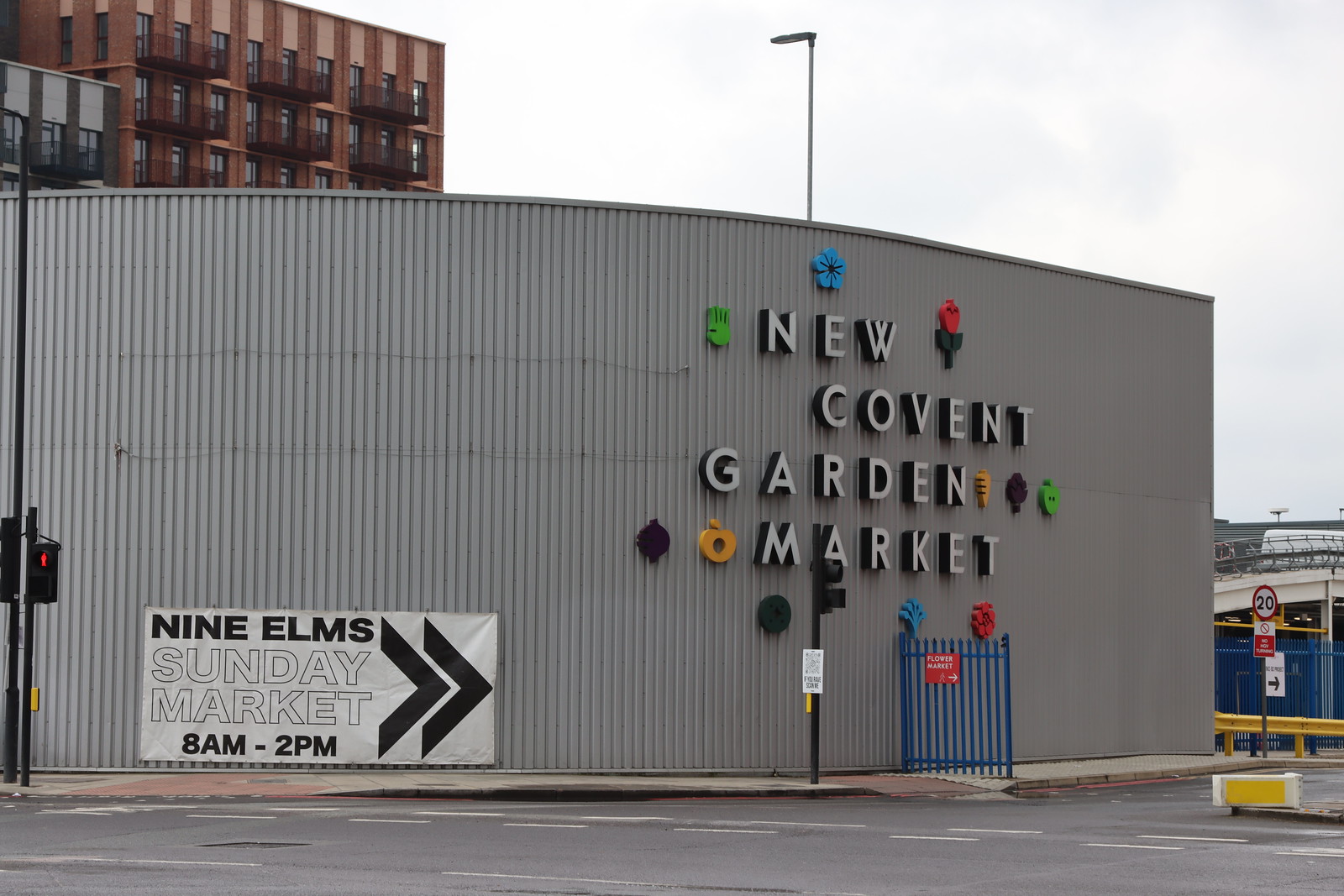This vibrant full-color photograph, taken outdoors on a cloudy day, offers a captivating glimpse of urban architecture and street life. Dominating the far upper left corner is a large building with multiple terraces and numerous windows, each featuring tiny decks. However, the height of the building remains indeterminate from this angle.

The focal point of the image is a distinctly curved metallic structure, gray in color, adorned with horizontal lines running the length of its visible surface. This building is identified as the New Convent Garden Market. Enhancing the urban scene, a couple of traffic lights are visibly stationed nearby.

Adding to the locale's character, a sign indicates the "9 Elms Sunday Market," specifying its operational hours from 8 a.m. to 2 p.m. and pointing to the right. The extreme right of the photograph reveals what appears to be a bridge. Near the building's side, there is a small, seemingly purposeless blue gate, injecting a hint of whimsy into the otherwise structured setting.